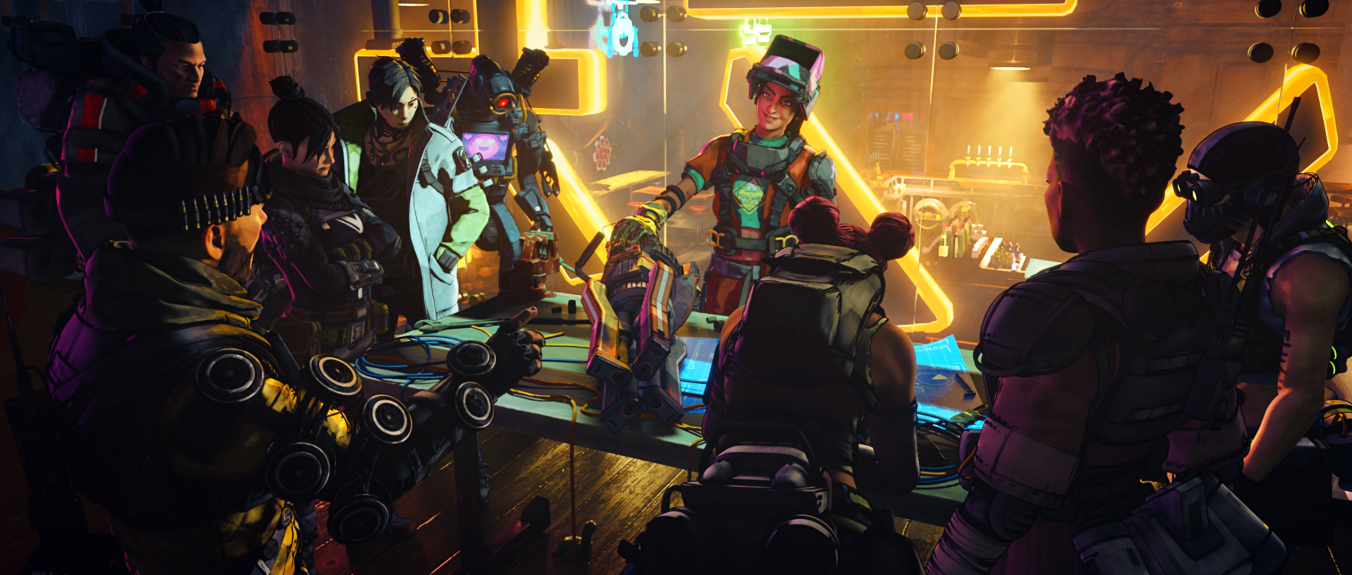The illustration depicts a cyberpunk-inspired interior, awash with vivid neon hues of yellow and green-blue, highlighting the scene with a saturated, futuristic glow. Set within what appears to be a dimly lit workshop or the back room of a club, a diverse group of heavily armored individuals and one identifiable robot gather around a large, metallic work table. At the table's center, a person with an orange jumpsuit adorned with belts and buckles stands out, sporting a flipped-up welder's mask that reveals their face. They are holding an intricate piece of machinery or armor, possibly a futuristic weapon. To the left, a character with bullets strapped between their hair and ear, wearing goggles, points towards the central figure, perhaps questioning or discussing something. Beside them, a woman with dark hair in a bun looks on with crossed arms, while another figure beside her in a thick jacket keeps their hand in a pocket. The background features large windows hinting at a well-lit area beyond, scattered with tables and bathed in dim neon light. The robot, with a screen displaying a mischievous smiley face, adds to the eclectic mix, reflecting the scene’s high-tech atmosphere. Over the table, a blueprint stretches out, and various figures, including females with cyberpunk attire and metallic gloves, are engaged in what seems to be an intense discussion or preparation.